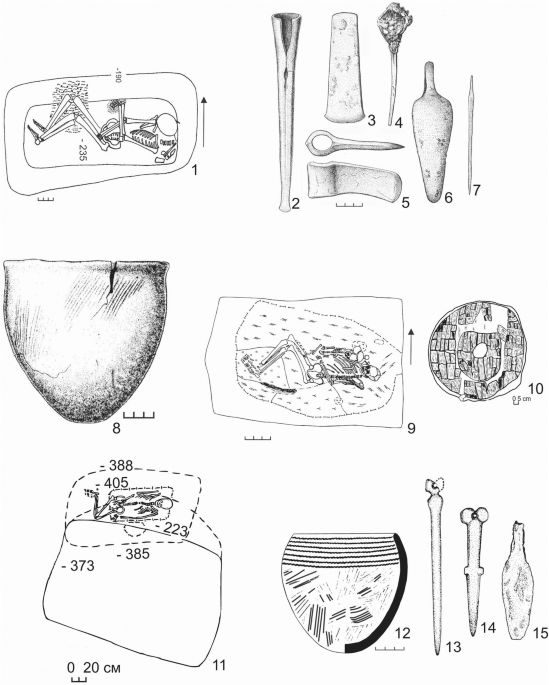This black-and-white sketch drawing comprises 15 numbered illustrations resembling those typically found in a detailed reference book. These pencil-like sketches are arranged in three rows within a vertically-oriented, white rectangle. The images display a variety of artifacts and tools, likely of archaeological interest.

Illustration 1, located in the top left corner, depicts a horizontal rectangle containing an indistinct mechanism with a circle and lines, paired with a human skeleton discovered with legs together and turned to the side. This skeletal depiction recurs in Illustration 9, showing consistency in archaeological finds.

On the right side, Illustrations 2 through 7 portray various tools and objects: 
- Number 2 is a cylinder, wide at the top and narrowing towards the bottom.
- Number 3 is cone-shaped.
- Number 4 features a stick with a flower-like end.
- Number 5 appears to be a scraping device.
- Number 6 resembles a vase.
- Number 7 is a simple stick.

Illustration 8 is a larger vase, while Illustration 10 is a circular drawing too ambiguous to identify clearly. Illustration 11 includes another skeleton. Number 12 depicts another vase, and the final set, numbers 13 through 15, represent additional old tools or artifacts similar in nature.

Overall, the sketches present a range of prehistoric items including bones, pottery, and tools, suggesting a careful study of archaeological discoveries.